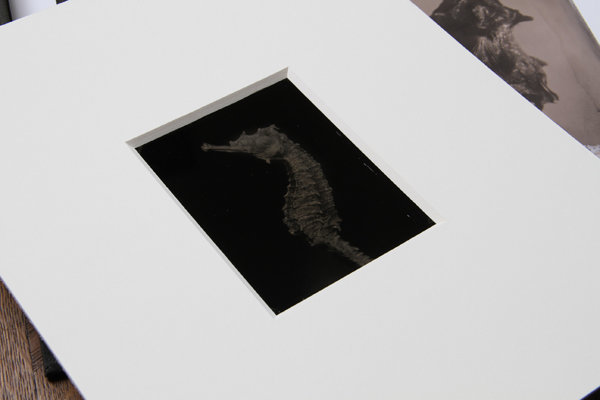The image features a rectangular, white-framed photograph laid diagonally on a possible wooden table, likely resembling an art studio or personal art room setting. The central photograph, framed in white, presents a striking black background with a detailed, gray seahorse in the middle. Off to the upper right, another barely visible photograph with a beige background displays a black and gray bird's head with a discernible eye and beak. There's no text present in the image, which captures an artistic and meticulous arrangement of photos viewed from a slightly left-angled perspective, suggesting someone is in the process of sorting or displaying valuable artwork or old photos.